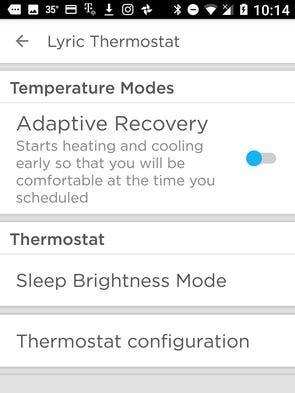A detailed screenshot of a phone app interface for managing a Lyric thermostat. The top of the screen includes a standard notification bar displaying the time, battery status, Wi-Fi signal strength, notifications from Messenger and Bluetooth, as well as icons for Photos, Instagram, Downloads, T-Mobile signal, email, and the current outdoor temperature. An arrow indicating additional icons that are not visible is also present.

Below the notification bar, the app clearly labels "Lyric thermostat," with an arrow pointing to the left. The main interface area is divided into several sections:

1. **Temperature Modes**: This section highlights various modes for controlling the thermostat settings.
2. **Adaptive Recovery**: Explains the feature that starts heating and cooling early to ensure comfort by the scheduled time, with an option to toggle this feature on or off.
3. **Time Schedule**: Provides options to schedule different temperature settings throughout the day.
4. **Thermostat**: Likely a main control or status display for the thermostat's current settings.
5. **Sleep Brightness Mode**: A setting for adjusting the display brightness when in sleep mode.
6. **Thermostat Configuration**: Allows for deeper configuration settings of the thermostat.

The overall layout has a clean white background with black lettering, some parts of which are bolder than others for emphasis. The bottom border of the interface is colored gray, providing a subtle framing to the app's display.

This app interface clearly focuses on providing an intuitive and comprehensive control over the Lyric thermostat, enabling users to efficiently manage their home's temperature settings.